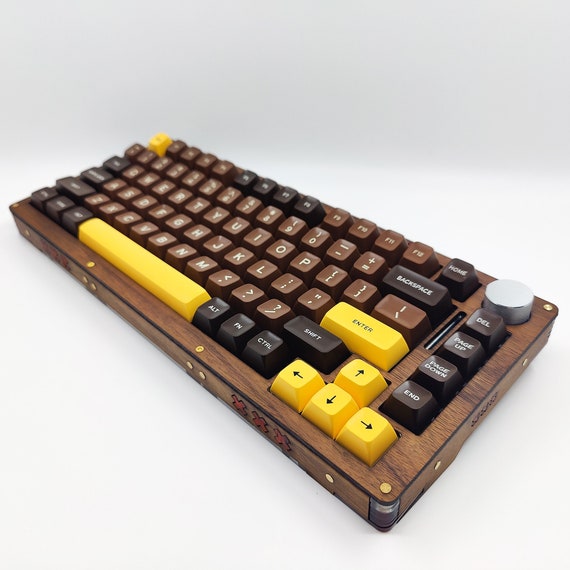The image showcases a close-up of a vintage-style keyboard with a distinct wood-like casing set against a varying off-white and gray background. The keyboard is diagonally angled from the upper left to the lower right, with a focus on the lower right, making the upper left slightly blurry. The keys display a blend of colors: the alphanumeric keys are brown, the function keys (such as Shift, Alt, and Control) are black, and the Escape, Spacebar, Enter, and arrow keys are yellow. Situated in the top right corner is a silver circular knob, and directly below it are the keys for Delete, Page Up, Page Down, and End. The design features raised buttons, exuding a retro aesthetic, and on the front flat part of the keyboard, there are three red X's. The image is devoid of any people or text, and the overall setting is bright, providing clear visibility of the detailed keyboard.